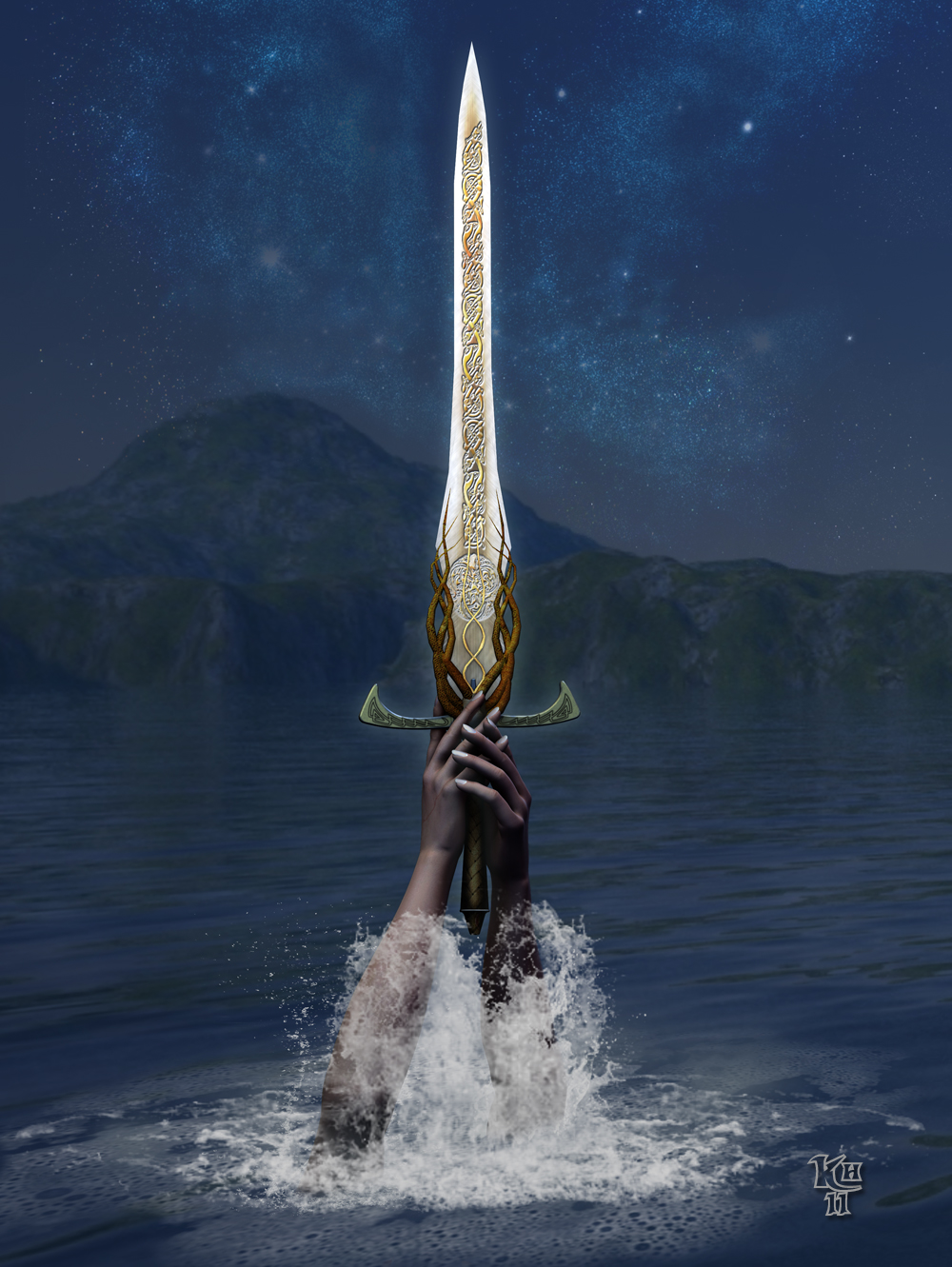In this captivating, computer-generated fantasy scene, a pair of pale, slender hands with white nail polish emerges dramatically from a serene, nighttime lake, water cascading off the forearms. The hands grasp an intricately designed sword that evokes myths like the tales of King Arthur and the Lady of the Lake. The sword itself features a silver blade adorned with Celtic runes and detailed gold engraving, complemented by bronze braiding along its edges and a golden hilt. Yellow vines entwine around a jade-colored section of the hilt, adding to its mystical appearance. In the background, a moss-covered mountain or hill looms under a star-studded sky, with the Milky Way galaxy faintly visible, creating a dreamy and magical atmosphere. Text marked "KH11" adorns the bottom right corner of this evocative portrait-oriented image.